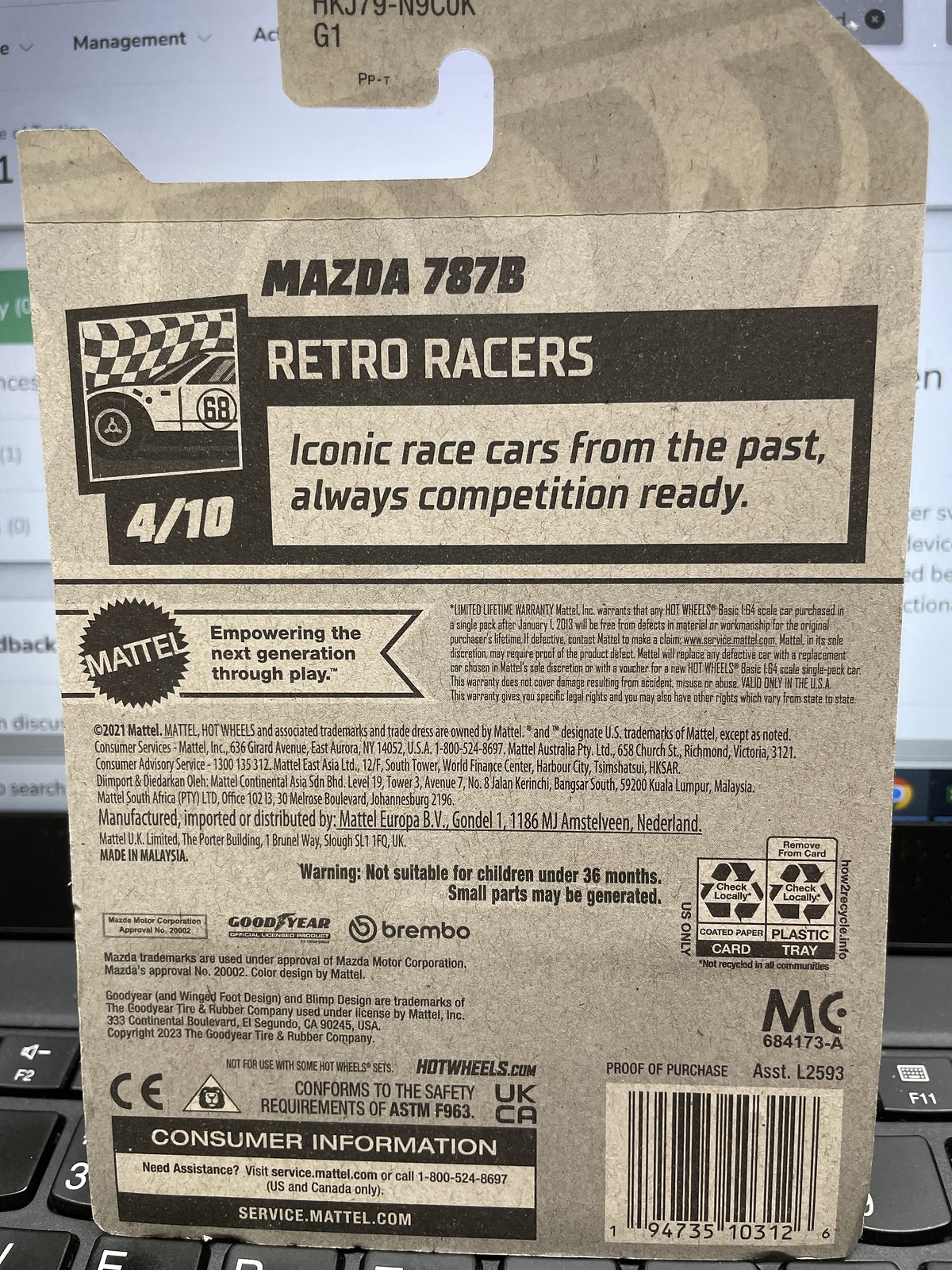This photograph captures the back side of a toy packaging, likely for a Hot Wheels or similar model, standing upright on a black laptop keyboard. The rectangular product cover, designed with a hook for hanging at the top, features a prominent green background. The title "Mazda 787B Retro Racers: Iconic race cars from the past, always competition ready" is boldly printed at the top, accompanied by a small graphic of a race car with a checkered flag, and the notation "4 of 10". The back of the packaging, made of a brownish, recycled material, below the main title, contains the Mattel logo along with a message stating "empowering the next generation through play." There's a plethora of smaller text including manufacturing, distribution, and consumer information, along with several icons. A barcode is located on the bottom right. In the background, the laptop screen is partially visible, indicating the device is on.